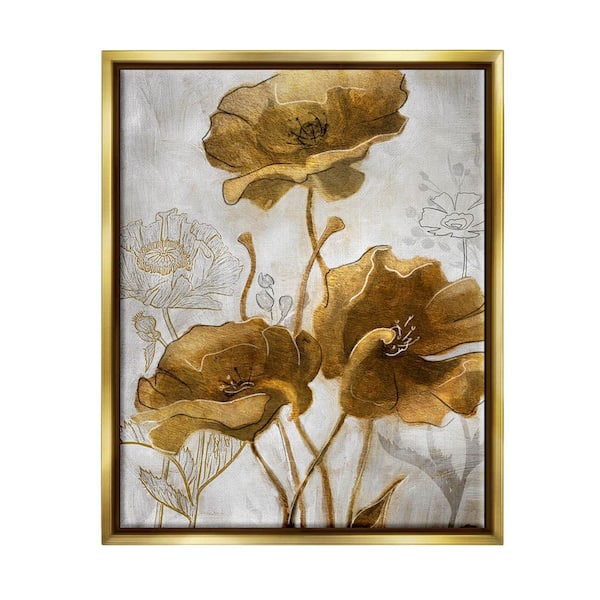The image is a painting or a digital artwork enclosed in a gold rectangular frame with a dark brown inset. The main focus is on three large, gold or golden-brown flowers with dark, withered stems, rising from the foreground. These flowers resemble roses or hibiscus, featuring detailed stamen and dark, crinkled petals that appear washed out, lacking vibrant colors. The background is predominantly white with a spray of black that gives a cloudy sky effect. Behind the main flowers, there are faint outlines of additional flowers and stems, rendered almost transparent with some outlined in gray and others in black and white lines, giving an impression of the flowers having their color faded or sucked away. This subtle detailing contrasts with the prominent golden-brown flowers in the foreground, contributing to the rustic and somewhat melancholic atmosphere of the artwork.